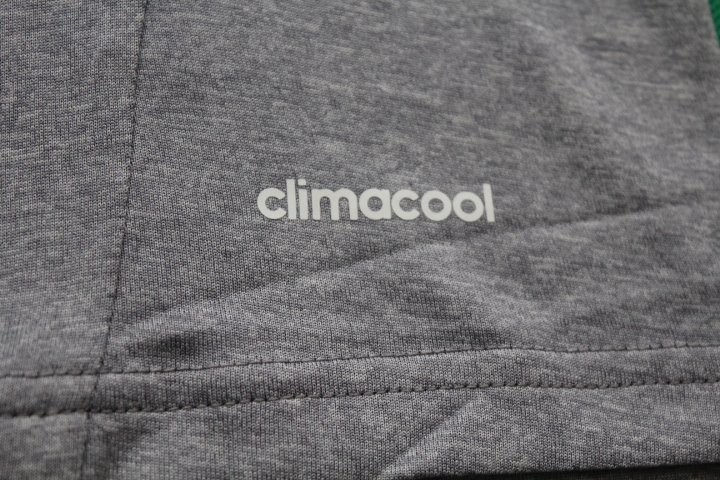This close-up photograph captures a section of a heather gray cotton clothing item, displaying a detailed view of its design elements. The focal point is a white, all-lowercase "climacool" logo imprinted on the fabric. The letters are crisply defined, with the text spelling out 'C-L-I-M-A-C-O-O-L' clearly discernible. The image is taken at such a proximity that the specific type of clothing remains indeterminate. Prominent in the composition are two visible seams: one vertical seam runs from the top to the bottom along the left side, while a horizontal seam approximately an inch from the bottom edge extends the entire width from left to right. The fabric features a diagonal crease starting from the middle of the right side and moving under the logo towards the vertical seam. Shadowing is noticeable towards the left, adding depth to the image, and subtle wrinkles in the fabric imply it is not lying completely flat, enhancing the texture and realism of the photograph.